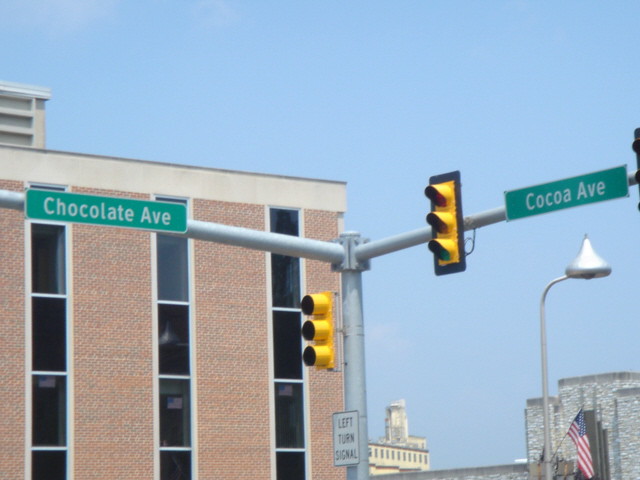The photograph captures a vibrant street intersection under a clear, blue sky, devoid of clouds. Dominating the center is a gray street light pole supporting two yellow traffic lights and street signs, which label the streets as Chocolate Avenue on the left and Cocoa Avenue on the right. Below the traffic lights, there's a sign indicating a "left turn signal." Adjacent to these, a metal bar extends outward with the street names inscribed on green rectangles with white text.

To the left, a tall, light brown building with three rows of multiple windows stretches upwards. An American flag is mounted on the wooden building to the far right, beneath another light pole that almost aligns with the flag. In the background, towards the upper right, stands what seems to be a clock tower, and nearby, a secondary light-yellow building is visible. The scene is filled with an assortment of details from the bustling streetscape, including the distinctive lamppost with a thin body capped by a small cone-like feature.